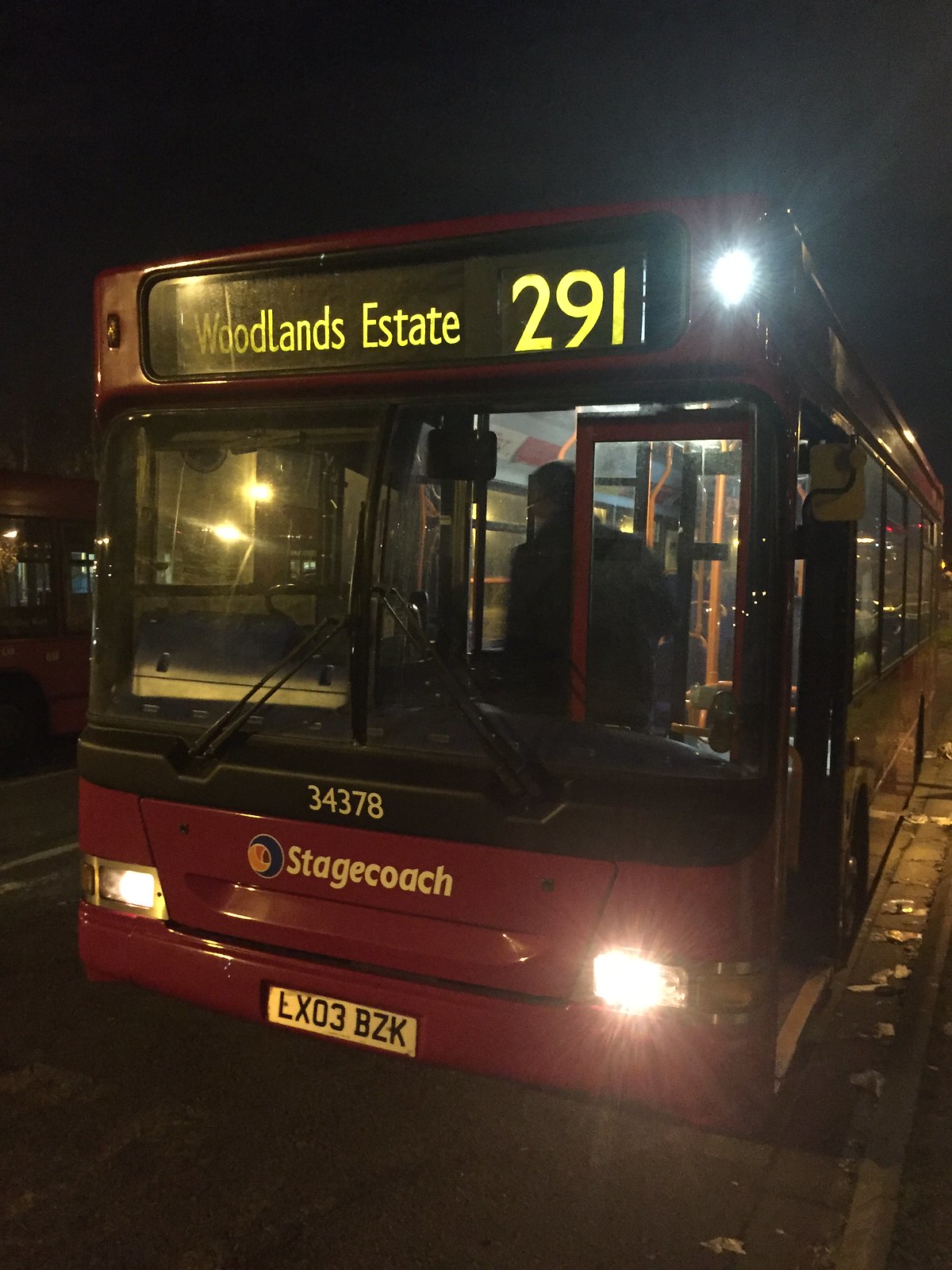The image is a detailed nighttime photograph of the front of a red Stagecoach bus, designated with the number 34378, as it stops on a dark street. Illuminated by its three functioning headlights—two at the bottom and one on the top right—the bus' destination display reads "Woodlands Estate 291" in bright yellow letters. Below the Stagecoach logo on the bus front, the license plate LX03BZK is visible. The bus's doors are open, revealing a person in a black coat, possibly a passenger or the driver, entering the vehicle. The street's dark pavement is discernible beneath and around the bus, adding to the overall nighttime urban setting of the scene.